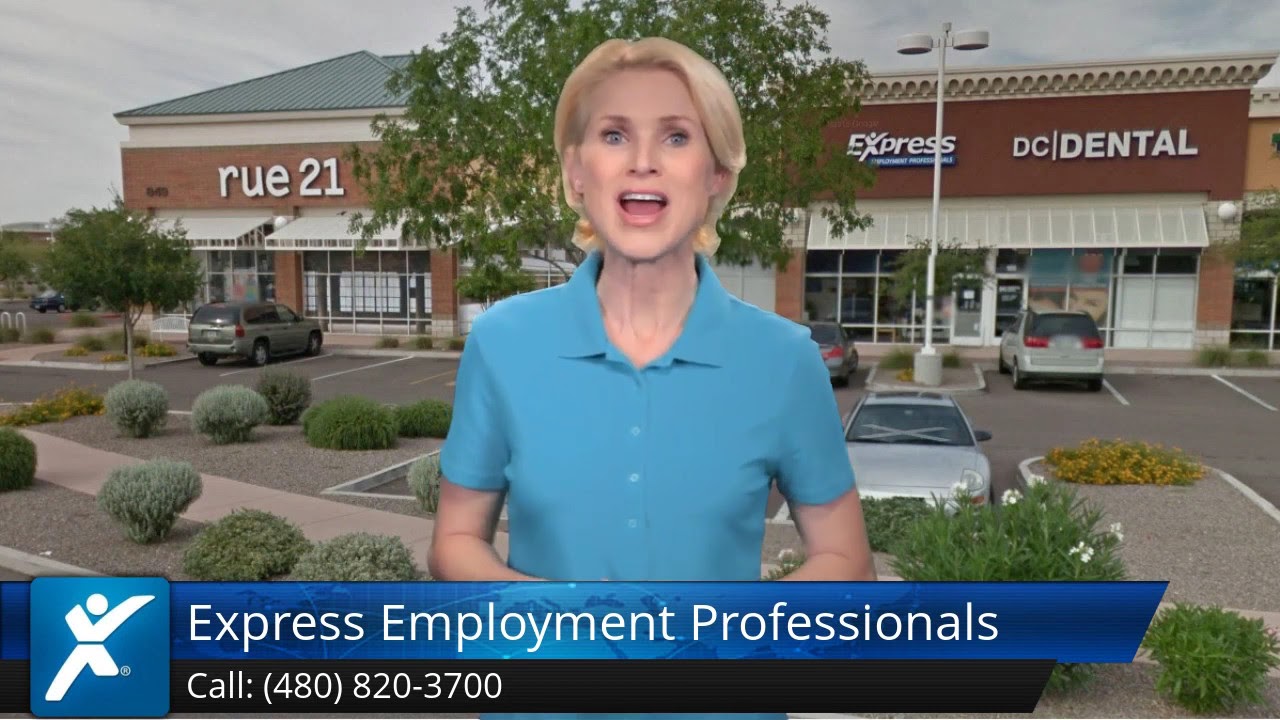The image appears to be an advertisement for Express Employment Professionals with the phone number 480-820-3700 prominently displayed at the bottom. It features a woman with blonde hair standing in front of a backdrop depicting a commercial area on a cloudy day. She is wearing a powder blue short-sleeved shirt and looks like she is speaking, suggesting the possibility of a video or a staged photo. Behind her are several stores, including Rue 21 on the left, Express Employment Professionals in the center, and DC Dental on the right, all located in a parking lot with multiple cars present. The surrounding environment hints at a deserty landscape with bushes and low vegetation.